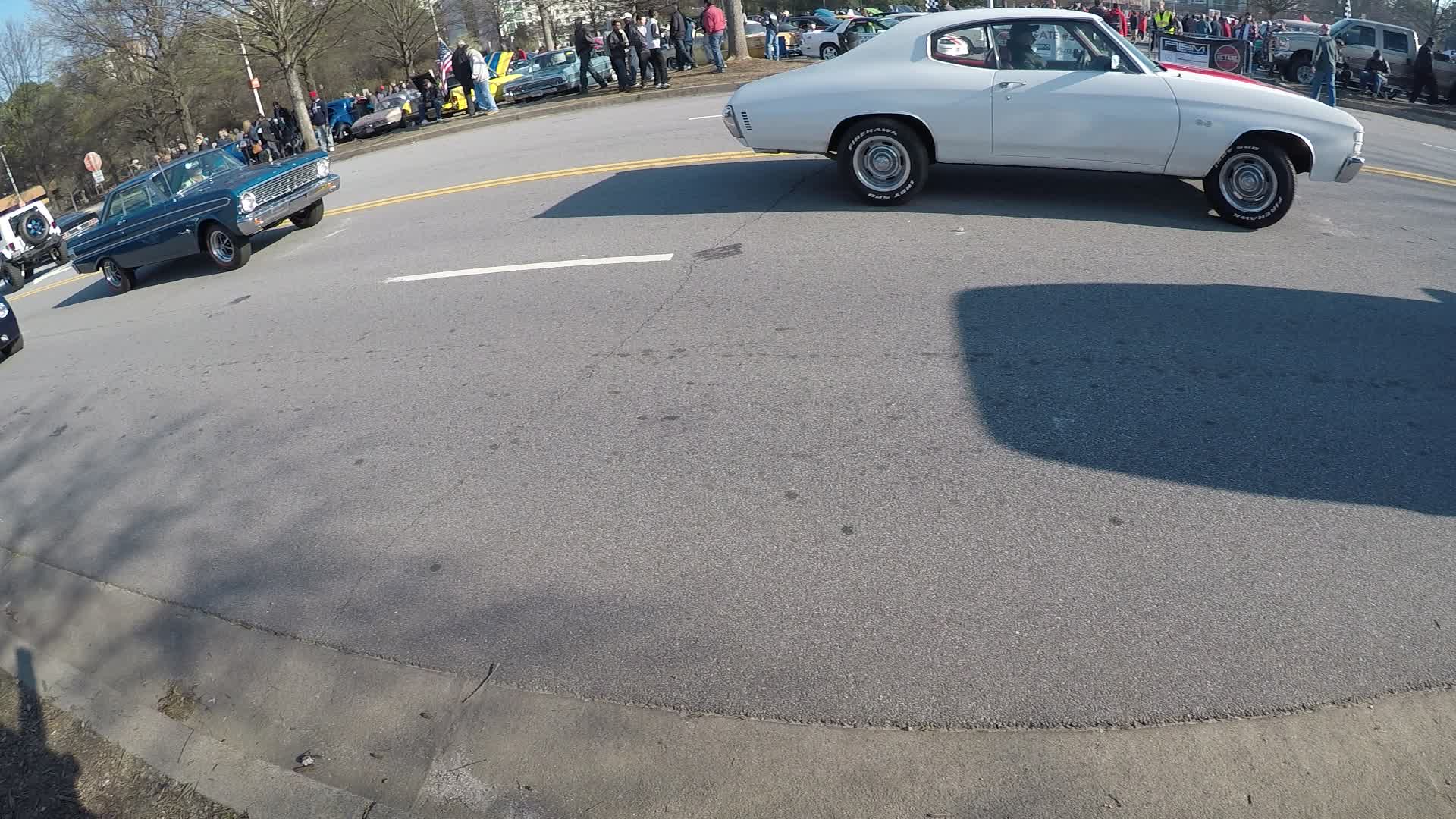This is a detailed color photograph, possibly taken with a fisheye lens, depicting a vibrant scene of a vintage car parade on a sunny day. The image shows a two-lane road, divided by a double yellow line, with classic cars traveling towards the right. Prominently in the foreground, there's a white car with elegant curves and white wall tires, potentially a Chevy Nova from the 50s or 60s. Following behind is a shiny blue-green sedan, likely a model from the same era, with an elongated profile.

On the opposite side of the road, people are gathered in a grassy area, enthusiastically watching the parade. Some are holding an American flag, contributing to a festive atmosphere that suggests a community event, possibly a vintage car show. The road itself is lined with dashed white lines and flanked by leafless trees in the background. Additionally, there is a newer model Jeep with a spare tire heading in the opposite direction, adding contrast to the scene filled with vintage charm. The shadows cast by the sunny weather enhance the nostalgic feel of this lively outdoor gathering.